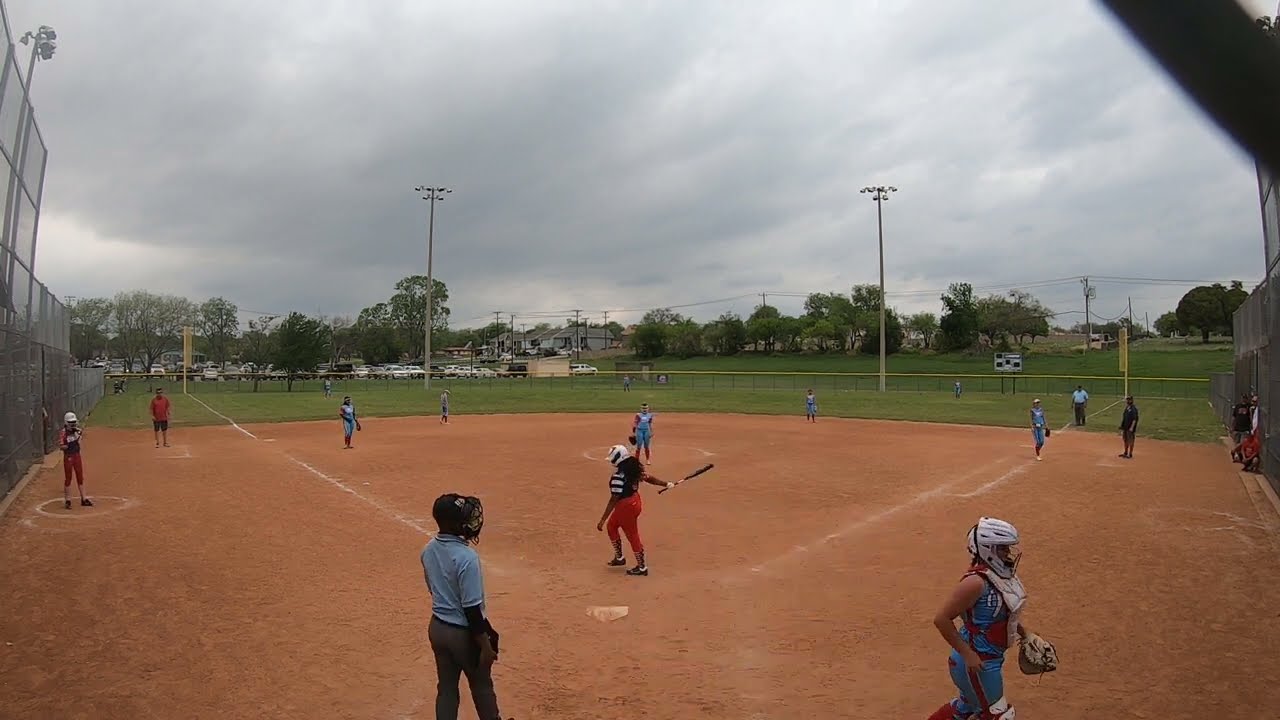This detailed image captures an outdoor baseball or softball game under a gray, cloudy sky. The scene is set on a dirt field with orange clay and distinct white lines forming a triangle, indicating the bases. Two key players are centered: one in a black t-shirt, black pants, and a white helmet standing at a base, and another in a blue uniform situated within a white circle, likely the pitcher's mound. The image hints at a mixed-gender game, with several players positioned around the field, some wearing helmets and others holding badges. In the far background, there's a lush green outfield and distant houses with a large parking lot full of cars. Tall light poles stretch towards the overcast sky, hinting at nighttime illumination, while trees and a fence line enclose the entire park. This expansive view appears to be taken from the perspective of a catcher, emphasizing both the immediate action and the broader, bustling park environment.